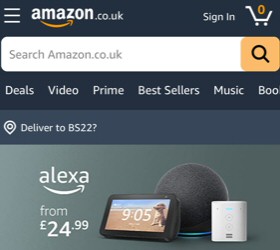The image is a graphic from a website, set within a square frame. The top section features a gradient background ranging from light black to medium dark gray. Against this backdrop, the text "amazon" is prominently displayed in bold, white, lowercase letters, with "co.uk" in smaller print beneath it. An orange arrow, resembling a smile, is positioned beneath the text.

To the right, the text "Sign In" appears, with the "S" and "I" capitalized. Adjacent to this is a white shopping cart icon, with the signature orange arrow integrated in the center.

Below this top section is a banner containing the search bar, which reads "Search Amazon.co.uk" in white text on a darker background. To its right, a black magnifying glass icon is set against an orange background.

Moving downward, the page lists several categories in white text: "Deals," "Video," "Prime," "Bestsellers," "Music," and "Books." Following this, a lighter gray banner displays the text "Deliver to BS22?" suggesting a location-based delivery option.

The bottom section features a graphic showcasing various Alexa products, accompanied by the text "Alexa from £24.99," with the British pound sign indicating the price.